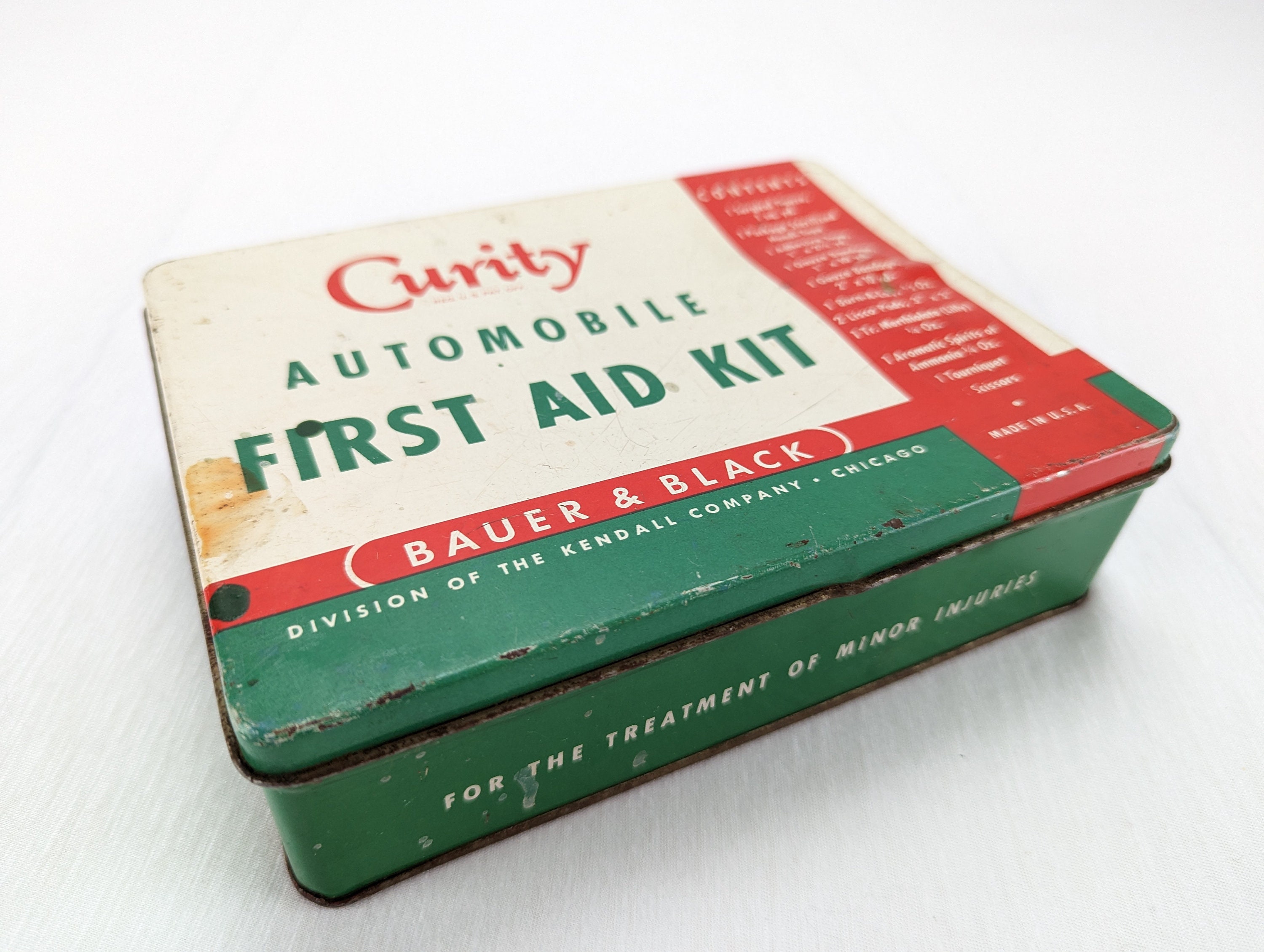The image depicts an old and worn metal first aid kit, likely made from tin, placed at an angle on a light gray or white textured table. The kit has a square shape with a thin profile, featuring rusted corners and numerous nicks in the paint but otherwise still in decent condition. The background is light-colored, complementing the aged look of the kit.

The top section of the first aid kit displays a white triangle in the upper left corner. Below this, in red letters, it reads "Cure-T," while beneath that, in green letters, it states "automobile" and "first aid kit." Farther down on the top cover, there's a label in white text that reads "Bauer & Black," enclosed in parentheses against a red background. Following this, with a green background as the base, it says "Division of the Kendall Company, Chicago."

On the right-hand side of the cover, a vertical red strip runs along its edge, containing small, somewhat blurred white writing detailing the kit's contents. The front face of the tin, primarily green in color, features additional white text that provides instructions for the "treatment of minor injuries." This meticulous detailing underscores the kit's original purpose and gives an authentic vintage charm to the well-preserved item.